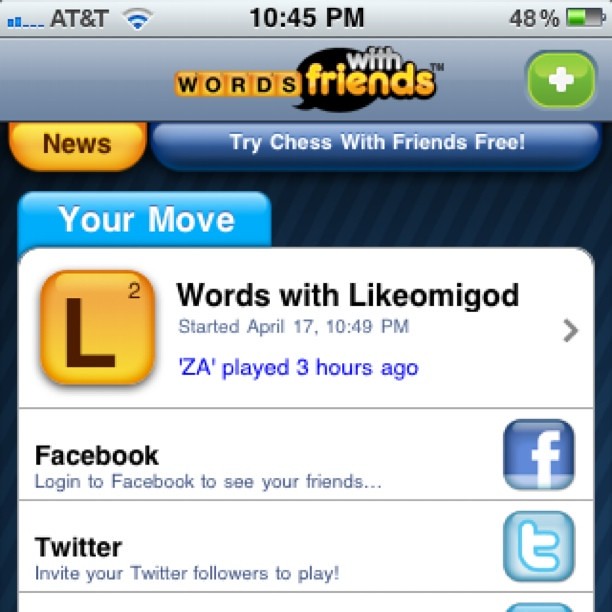This screenshot captures the top portion of a Words with Friends game on someone's phone. At the very top, the gray status bar displays the phone carrier (AT&T), the time (10:45 PM), the battery life (48%), and the signal strength (two out of five bars). Below this, centered, is the Words with Friends icon, featuring the word "Words" on yellow squares with black letters, and "Friends" on gold with "with" in white above it and a black speech bubble behind. To the right of this icon is a green square with a white plus sign. 

Directly beneath this icon row, a yellow bubble reads "News", and a blue bubble states "Try Chess with Friends Free!" in white letters. Further down, a blue tab on the left declares "Your Move!" in white text beside a gold beveled square with the letter "L". To its right are the words "Words with Like, Oh My God!" in black print on a white background, alongside additional details such as "Started April 17th, 10:49 PM" and "Z.A. played three hours ago" in blue print.

At the bottom portion of the screenshot, there are options to log in via Facebook or Twitter, each accompanied by their respective logos and brief descriptions for connecting or inviting friends through these social media platforms.